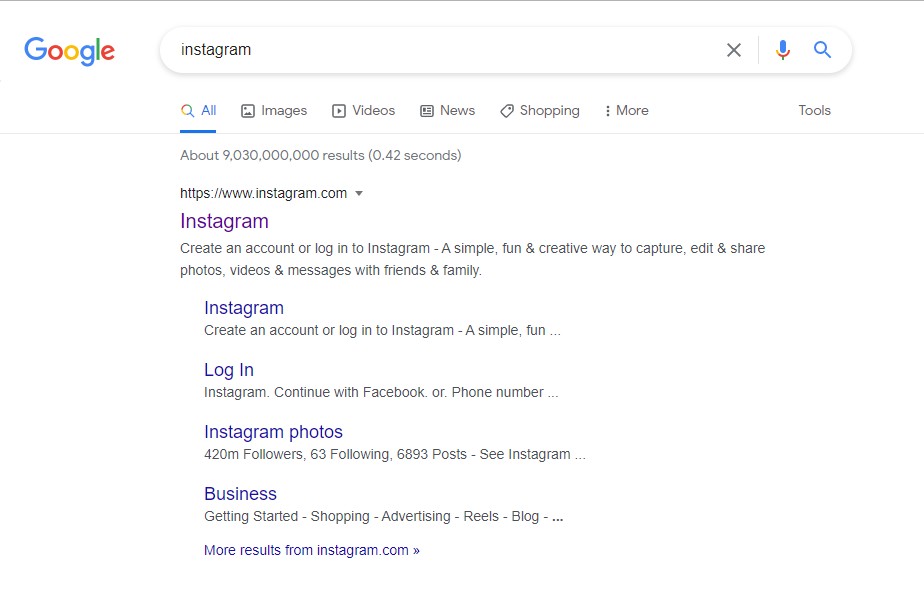This screenshot captures a Google search results page for the query "Instagram." 

In the top left corner, the iconic Google logo is prominently displayed, rendered in its characteristic font with colors alternating between blue, red, yellow, blue, green, and red. Below the logo, the search bar contains the term "Instagram," indicating the user is seeking information or services related to the social media platform.

Immediately underneath the search bar, a navigation menu offers additional search categories: All, Images, Videos, News, Shopping, More, and Tools. The results suggest there are approximately 9,030,000,000 entries, with the search completed in 0.42 seconds.

The first result displays the official Instagram URL (https://www.instagram.com) and a brief description: "Instagram. Create an account or log into Instagram. A simple, fun, and creative way to capture, edit, and share photos, videos, and messages with friends and family."

Following this, the page lists options for account management, including "Create an account or log into Instagram" and "Log in." Additionally, information is provided about Instagram's various features and services, including the ability to continue with Facebook or via phone number.

Further results include brief data about Instagram's profile, highlighting its 420,000,000 followers, 63 following, and 6,893 posts, along with links to sections such as Business, Getting Started, Shopping, Advertising, Reels, and Blog.

It is worth noting that the image is devoid of any photographic or illustrative content, consisting solely of textual information.